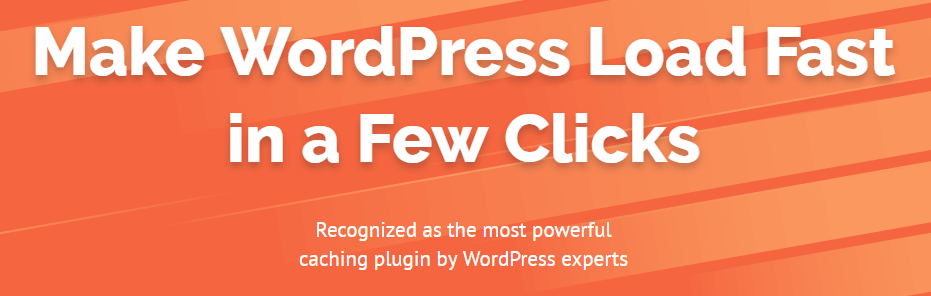The image features a bold orange background with lighter orange bars extending from the upper left corner to the bottom right, gradually fading as they descend, giving a textured appearance. At the top center of the image, large white text reads, "Make WordPress Load Fast." Directly below this, center-justified, smaller white text proclaims, "In a Few Clicks." At the bottom of the image, a smaller white font states, "Recognized as the most powerful caching plugin by WordPress experts."